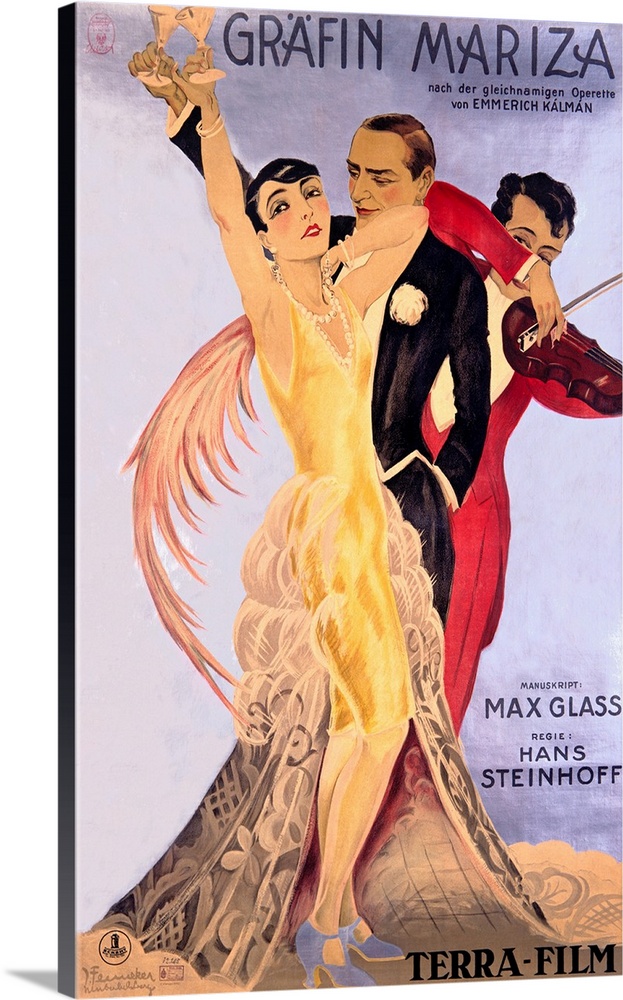The image is a vertically rectangular, multi-color print piece, likely from a book or magazine cover. The left side of the image features a simple border, which is the spine of the book, while the background is predominantly bluish with a small shadow in the lower left-hand corner. Across the top, in black or dark blue font, the text reads "Grafen Marisa." Below this, additional German text is present but not fully legible. On the lower right-hand corner of the cover, the names "Max Glass" and "Hans Steinhoff" are visible, along with "Terra Dash Film" at the very bottom.

The central illustration depicts three characters styled in a 1920s aesthetic. In the foreground, a woman dressed in a luxurious yellow dress and adorned with a pearl necklace is holding a martini glass aloft, her pose directed towards the viewer. Behind her, a man in a black suit with a white boutonniere also raises a glass, his gaze fixed on the woman. Further in the background, another man dressed in a red suit is seen playing a violin. This vibrant scene captures a sense of celebration or an elegant gathering. The overall design and illustration emphasize the opulent and artistic style of the 1920s.